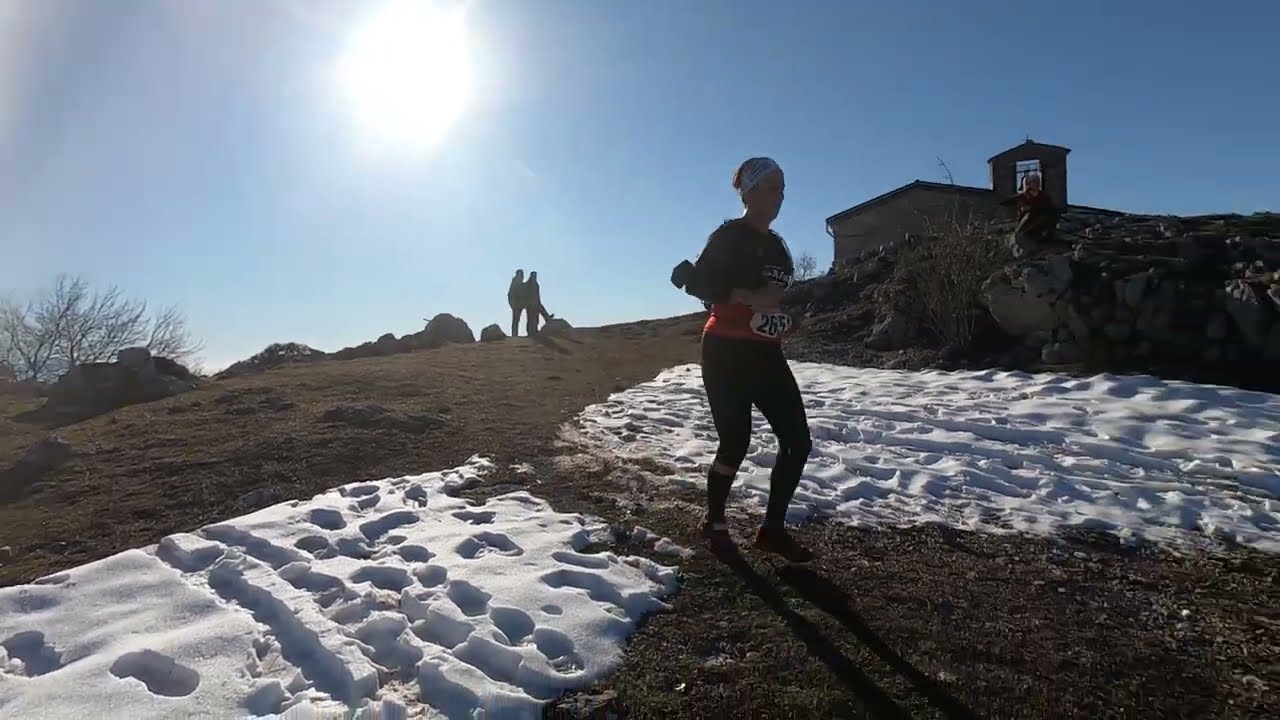The photograph captures a dynamic outdoor scene on a bright, sunny winter day. The image centers on a woman, likely participating in a marathon, as indicated by her attire: a black shirt with a red waistband, displaying the race number 265 in black numbers inside a white circle. She wears a white bandana and black leggings. The woman is running downhill through a barren, dirt-covered path flanked by patches of snow, which are heavily trodden with footprints and tire tracks.

The landscape features a steep incline stretching from the left to the right. In the background, there is a clear blue sky with a large, radiant sun positioned near the left-hand corner, casting long shadows. To the right, the top of a building, possibly a church or hacienda with a small bell tower, rises against the horizon. Silhouetted at the crest of the hill, slightly left of the center, stand two people watching the runner as she descends. The scene is set in a rural, wintry area, suggesting that it could be located in Spain or New Mexico, due to the architectural hints.